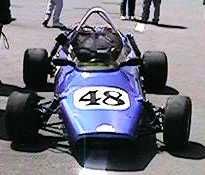This image features a small, open-wheel Terrapin racing car, showcasing a bright bluish-purple color with a distinctive white circular design on its torpedo-shaped body, prominently displaying the number 48 in jet black. The car is notably flat, with black wheels extending higher than the body, and equipped with a double wishbone suspension on the front. Above the driver's small black seat, a metal roll bar ensures safety. Positioned on an asphalt road with white dotted lines, the backdrop includes the partial view of people's legs, likely spectators or participants, cut off at the top of the image. Additionally, some camera equipment can be seen peeking through the top left corner, hinting at a possible photo or video shoot in progress.